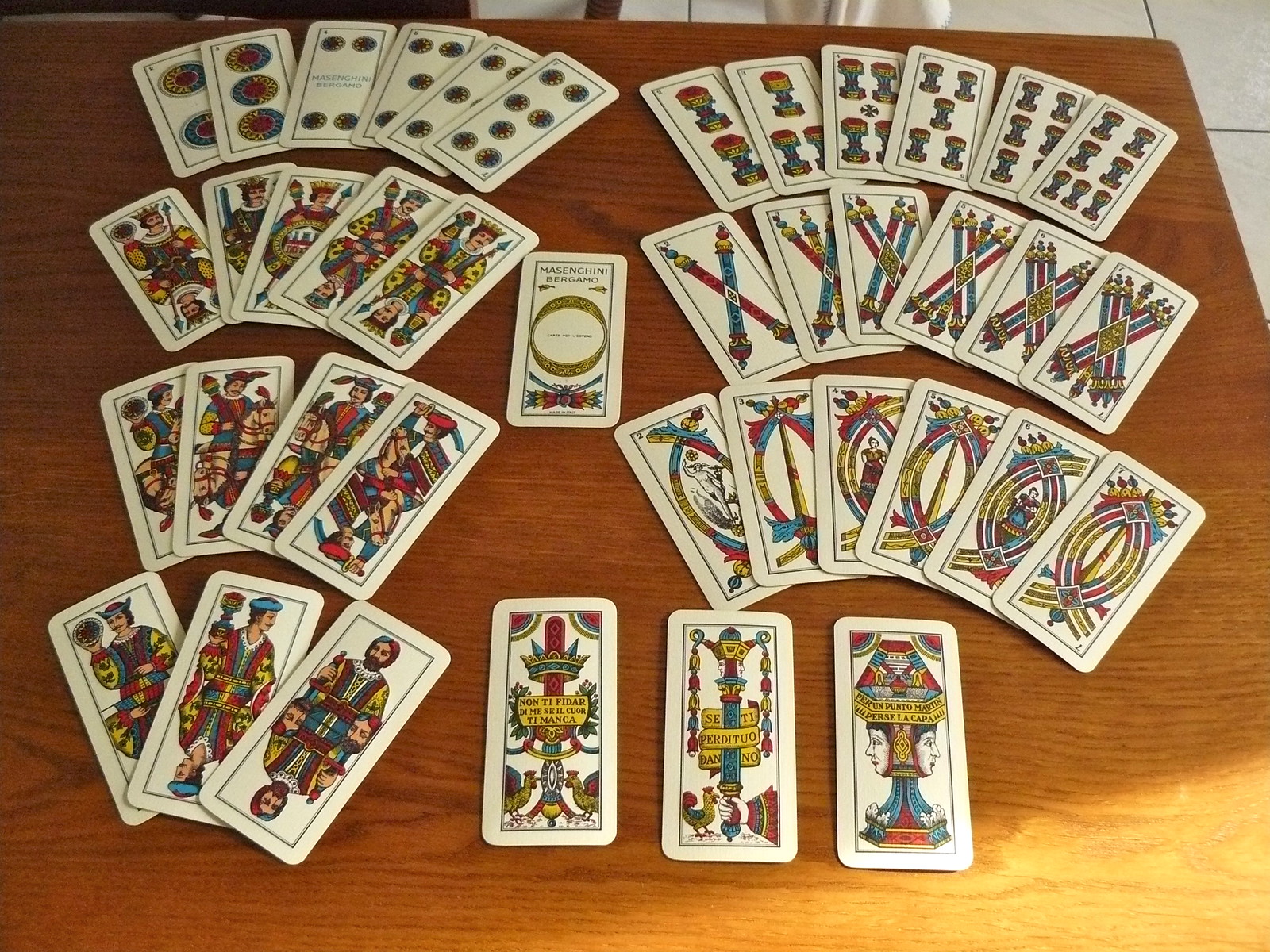This photo captures an intriguing and richly detailed setup of unusual cards spread across a wooden table. The image is shot from a steep angle, roughly around 70 to 80 degrees, allowing for a comprehensive view of the arrangement. The table's wooden surface is clearly visible, showcasing its light and dark brown grain patterns. A shadow obscures most of the tabletop, leaving only the bottom right corner brightly lit. 

The cards in the photo deviate from typical playing cards; they are notably long and narrow, significantly more rectangular and taller. Approximately 30 to 40 cards are distributed across the table in a somewhat organized yet artistic manner. On the left side, the cards are arranged in descending rows: the top row has six cards, the next has five, followed by rows of four and then three cards. These cards overlap at the bottoms but fan out at the top, displaying their design. 

In the center of the table lie two solitary cards, isolated from the grouped formations but equally ornate. The right side mirrors the left, beginning with a row of five cards, also fanned out meticulously.

The cards boast vibrant and ornate illustrations with an array of colors such as reds, greens, yellows, golds, and blues. Imagery on the cards includes noble figures adorned in traditional attire, sometimes mirrored to create a symmetrical effect. Other cards feature crossed swords in varying quantities, suggesting elements of a game or symbolic representation.

Beneath the table, a white tiled floor is faintly visible, hinting at a continued space beyond the wooden surface. An indistinguishable object appears near the edge of the image, adding an element of curiosity to the scene.

This captivating arrangement of cards and the interplay of shadow and light combine to create a visually stimulating and intriguing composition.